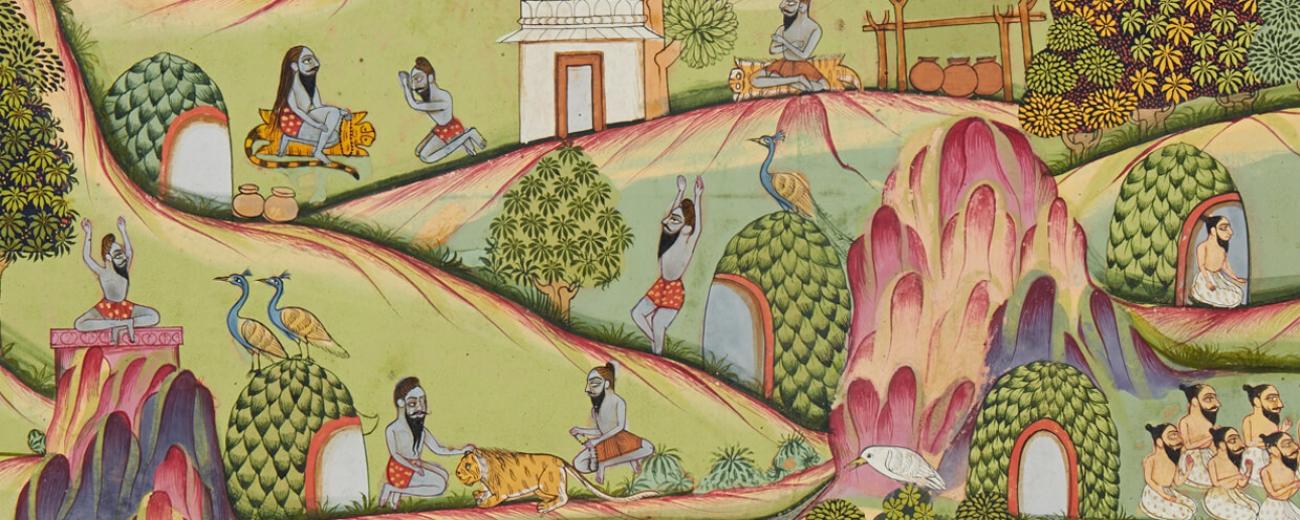This intricate painting presents an outdoor scene filled with a variety of elements that collectively create a sense of serene, possibly Eastern religious practice. The image is saturated with lush greenery and vibrant colors including various shades of green, yellow, pink, blue, orange, white, black, brown, beige, and peach. 

In the bottom right corner, there are five people kneeling and praying. Above them, nestled within a hut, a person sits in a meditation pose, surrounded by plants. To the immediate left, a dense bush occupies the space. Central to the composition, a person practices yoga next to a bird, while the bottom left showcases additional birds and people engaged in their activities. 

The top left corner features more huts, a tiger, and several more people interacting within the scene. The upper part of the image displays another individual, seemingly seated on an animal with a tail, further adding to the mystical quality of the artwork. Scattered throughout the scene are trees, including large bushes, rolling hills, and a plethora of birds, peacocks, and other flora, contributing to the rich tapestry of natural and human elements.

Overall, the piece resembles a mural or detailed graphic print, characterized by its colorful and methodically placed objects, revealing a peaceful tableau of people in various states of worship and contemplation amidst nature's bounty.